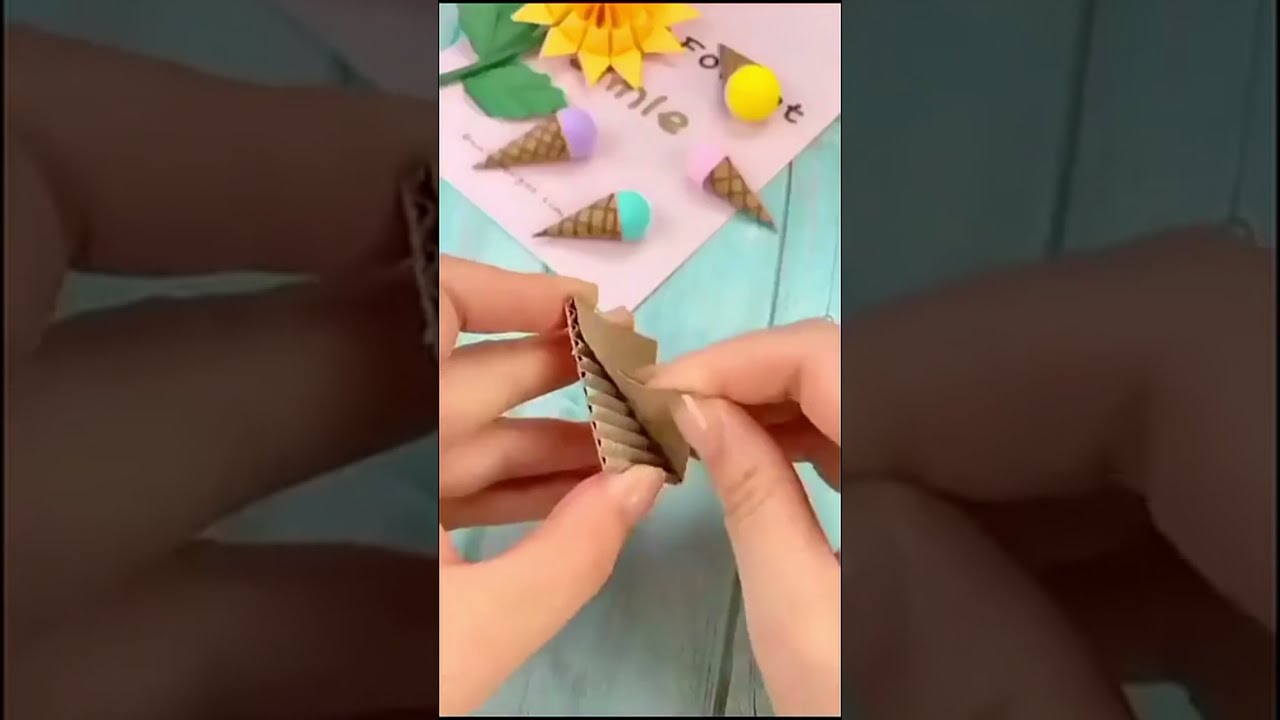In this detailed still from a TikTok video, a woman's hands with pale skin are captured in the process of peeling apart a small section of corrugated cardboard, revealing its bumpy interior layer. The scene is set on a blue wooden table with a pink piece of paper lying beneath her hands. Around her, a collection of intricate craft projects can be seen, including a meticulously crafted yellow paper sunflower with green leaves and several three-dimensional miniature ice cream cones made from brown paper adorned with dark markings. Each cone features a scoop of pastel-colored "ice cream" in shades of light lavender, teal, pink, and yellow, possibly made from cotton balls. This central image is framed by a wider border on the left and right sides, constructed from zoomed-in, dark-tinted versions of the same main picture, creating a portrait-like appearance in landscape orientation.